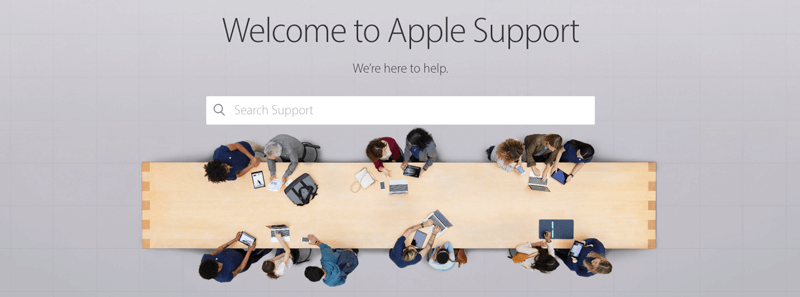This horizontal rectangular image is a detailed screenshot of an Apple Support web page. The top of the page prominently features the text "Welcome to Apple Support" in bold, large font, immediately followed by the smaller text, "We're here to help." Below this welcoming introduction is a conspicuous white search bar marked with a gray magnifying glass icon, where faint gray text prompts users to "Search Support."

The background of the entire webpage is a subdued gray, providing a subtle contrast to the black text and the white search bar. Positioned below this interface, the image transitions into a photograph of a work table, captured from an overhead perspective, as if the camera were fixed on the ceiling. 

This pale, butcher-block-style wooden table spans the width of the image, forming a prominent horizontal band. Gathered around the table, fourteen people are engrossed in various tasks, divided evenly with seven on the top side and seven on the bottom. The individuals are engaged with an array of Apple devices, including laptops, tablets, and phones, creating a dynamic scene of collaborative activity and technological engagement.